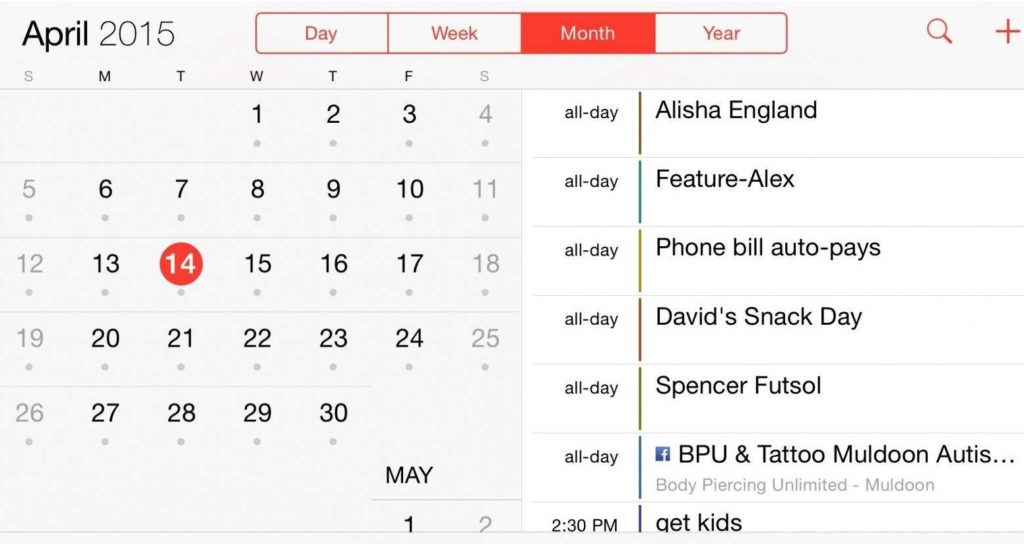Here is a detailed and cleaned-up descriptive caption based on the given image:

On a light gray background, the top left corner features the text "April 2015." The central part of the image is divided into four sections labeled "Day," "Week," "Month," and "Year," presented in a single rectangular line. The "Month" section is outlined in red. Below these sections, a calendar is displayed for April 2015. The days are organized so that the month starts on a Wednesday, April 1st, and ends on Thursday, April 30th. Notably, April 14th is highlighted with a red circle and white text. Under the April calendar, the first two days of May are visible and labeled.

To the right of the calendar, there are seven columns, each marked with the label "All Day," except for the bottom row which specifies "2:30 p.m." The entries in each row from top to bottom are as follows:
- Alicia England
- Fisher - Alex
- Phone bill auto pays
- David snack day
- Spencer futsal